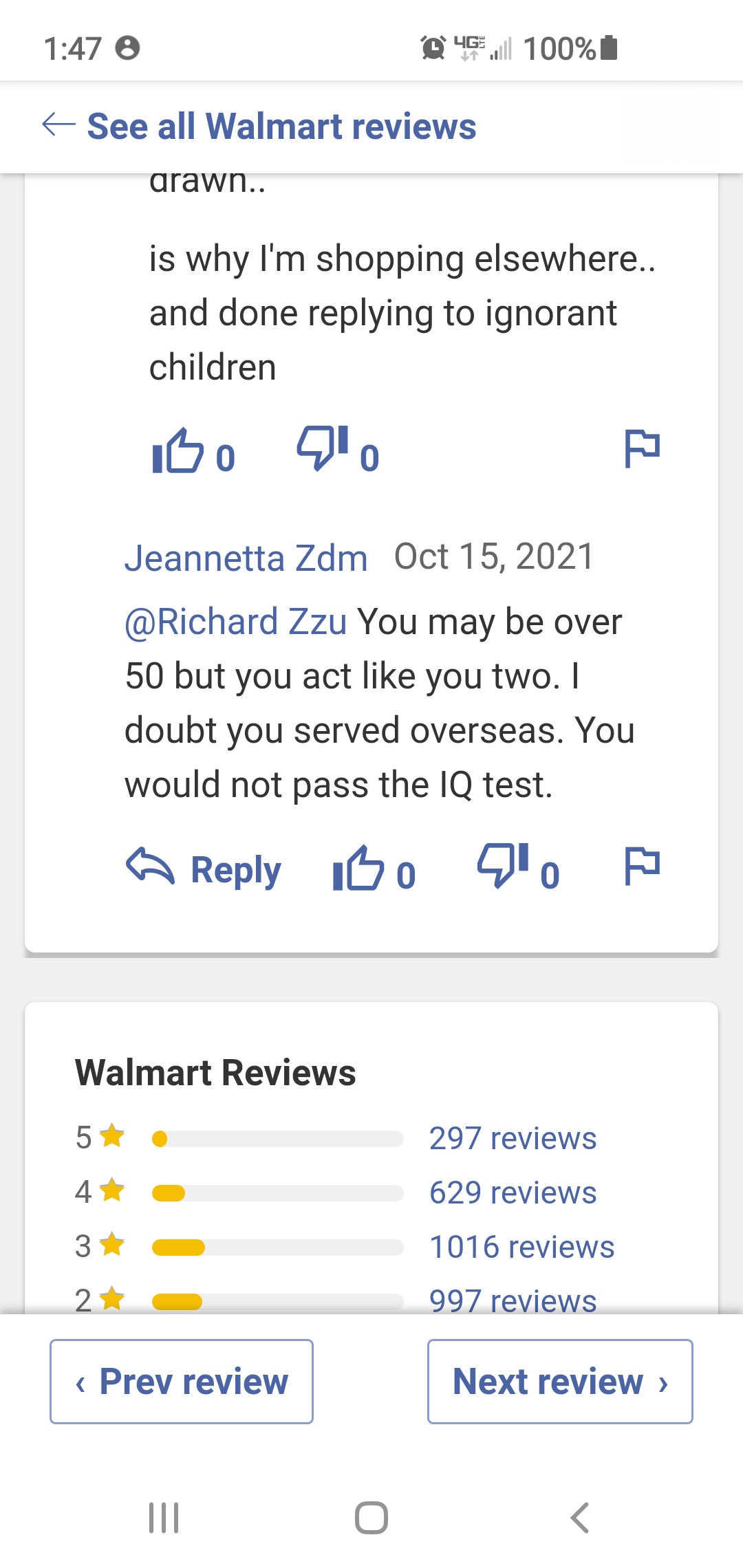This image is a cell phone screenshot of a Walmart Reviews page, captured on October 15, 2021. The screenshot shows a snippet of communication between users, with the username "Janetta SDM" being notably visible. The beginning of Janetta's post is cut off, but it begins with the word "drawn" and concludes with the statement "is why I'm shopping elsewhere and then replying to ignorant children." This message has been given the option to receive thumbs up or thumbs down votes, both currently at zero.

The screenshot also captures a message addressed to user "Richard ZZU," stating: "You may be over 50, but you act like you too. I doubt you served overseas. You would not pass the IQ test." This harsh reply has similarly available options for thumbs up or thumbs down, both also at zero.

At the bottom of the screenshot, the "Walmart Reviews" section showcases aggregated star ratings. The reviews are categorized as follows: 997 two-star reviews, 1,016 three-star reviews, 629 four-star reviews, and 297 five-star reviews. Navigation options are provided to preview either the previous review using a left arrow or the next review using a right arrow.